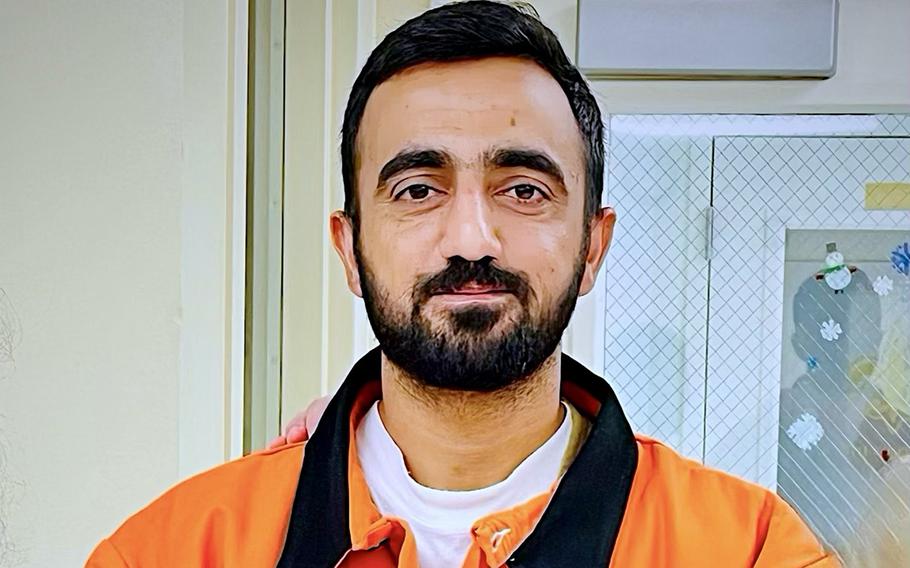The image portrays a close-up of a man with olive-toned skin, possibly of Middle Eastern descent, looking directly into the camera. He sports short, neatly combed black hair, bushy black eyebrows, and a full beard that extends onto his neck, complemented by a thick mustache. The man is wearing a white T-shirt beneath an orange jacket with a black lapel. On his right shoulder, the fingers of an unseen individual are visible, suggesting someone's presence just outside the frame. Behind him is a cream-colored wall and a door featuring wire mesh embedded within its glass. The window on the door displays stickers of snowflakes and a snowman, and it reflects the back of the man's head. The overall scene evokes a setting that could be akin to a school or an institutional building.